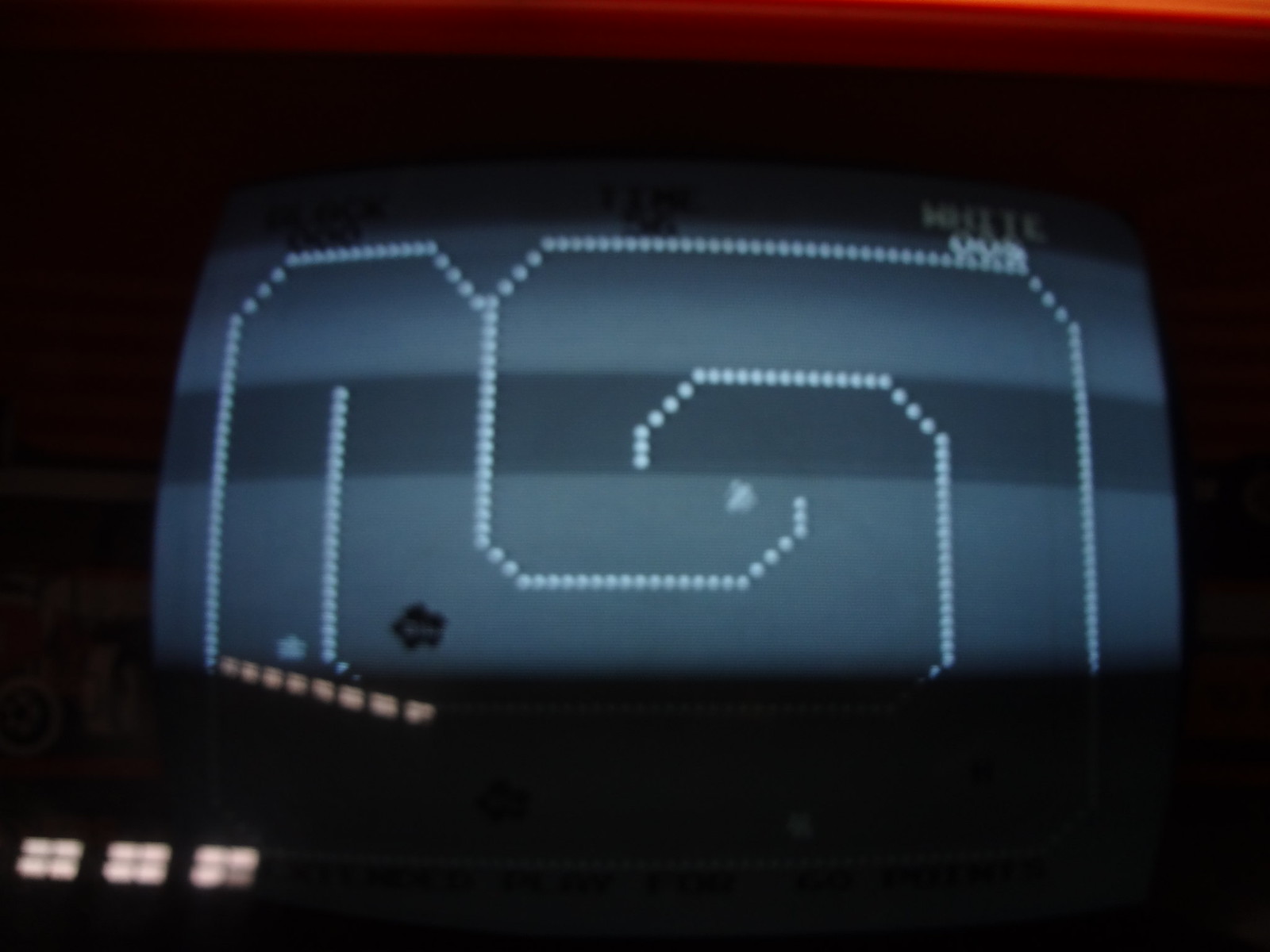This close-up image captures the vintage essence of an old arcade game from the late 1970s to early 1980s. The visual is tightly focused, revealing only the interior black framework and the reflective glass encasing the monitor. Through the sheen of the glass, the monochromatic game screen comes into view, dominated by shades of gray, white, and black, indicative of a very early racing game. Simplistic in nature, the screen features rudimentary graphics, including a small black blob resembling a race car and dashed lines suggesting the racetrack boundaries. In the top right corner, there are faint, white symbols or text that appear to be “YY” or similar markings. The ambient reflections of lights on the glass hint at the arcade setting, reminiscent of classic entertainment venues such as a mall or an ice cream shop. The overall composition evokes a strong sense of nostalgia for the archaic yet charming gaming technology of a bygone era.